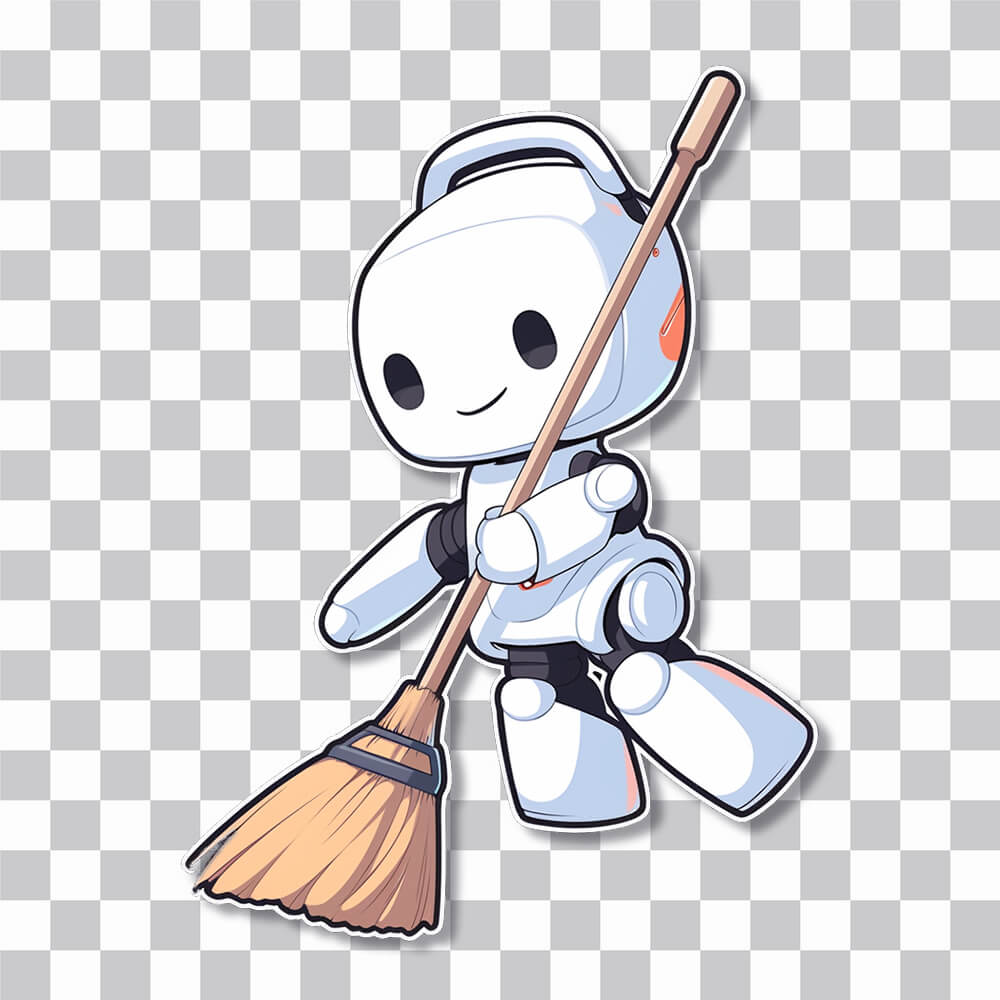This is a detailed graphic illustration of a charming robot, reminiscent of a snowman, set against a checkered background of gray and white squares. The robot, primarily black and white, features a body shape akin to a lunch pail or snowman, with a cylindrical form that extends into a nearly circular head. It has black electronic arms attached to its body with black joints, leading to white hands that lack fingers. The robot’s face displays expressive black eyes and a small black smile, giving it an endearing appearance. Perched atop its head is a distinct handle. In its left hand, the robot grips a light brown broom halfway up the handle, with bristles matching the same brown hue and encircled by a thin metal strip near the base. This scene, framed like a sticker design, emphasizes the robot’s domestic task and could easily be envisioned as a fun character in a game or a design for printable merchandise.